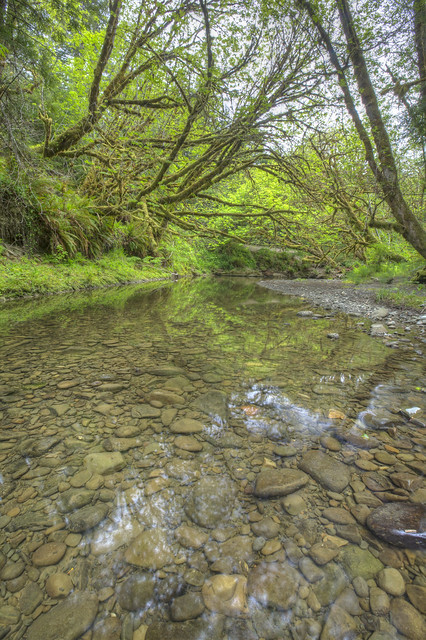This photograph captures a tranquil, shallow stream running through a secluded, natural landscape. The stream's clear water reveals a variety of tan and brown rocks scattered on the bottom. The water also reflects the surrounding environment, including a very light blue sky and lush trees that border both sides of the stream. The trees, displaying vibrant green and brown hues, arch towards the center, creating a picturesque canopy. The grassy and bushy banks of the stream add to the verdant scenery, with pebbles of various sizes visible along the water’s edge, and a notably large brown pebble situated at the bottom right of the frame. Overall, this serene and remote setting is accentuated by the clear reflections on the water's surface, highlighting the natural beauty of the scene.